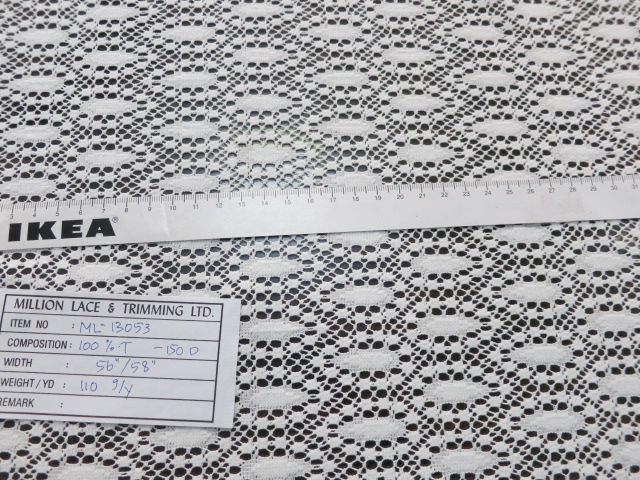The black-and-white photograph displays an entire lace doily that extends beyond the image's edges. The intricate lace features oval designs outlined in black with a light-colored interior. Across the midsection of the lace is a white measuring tape bearing the IKEA logo in large black letters, extending off the image's left and right sides and marked in centimeters. In the bottom left corner of the image, there is a small white card with a black rectangle at the top, labeled "Millian Lace and Trimming Ltd." The card is organized into six boxes that provide detailed information about the lace: the item number, composition (100% of an unspecified material), width, weight per yard, and a section labeled "Remark," which appears to be blank. The inclusion of the measuring tape and the detailed card suggests that the lace is being measured and documented for purchase, possibly at an IKEA store.